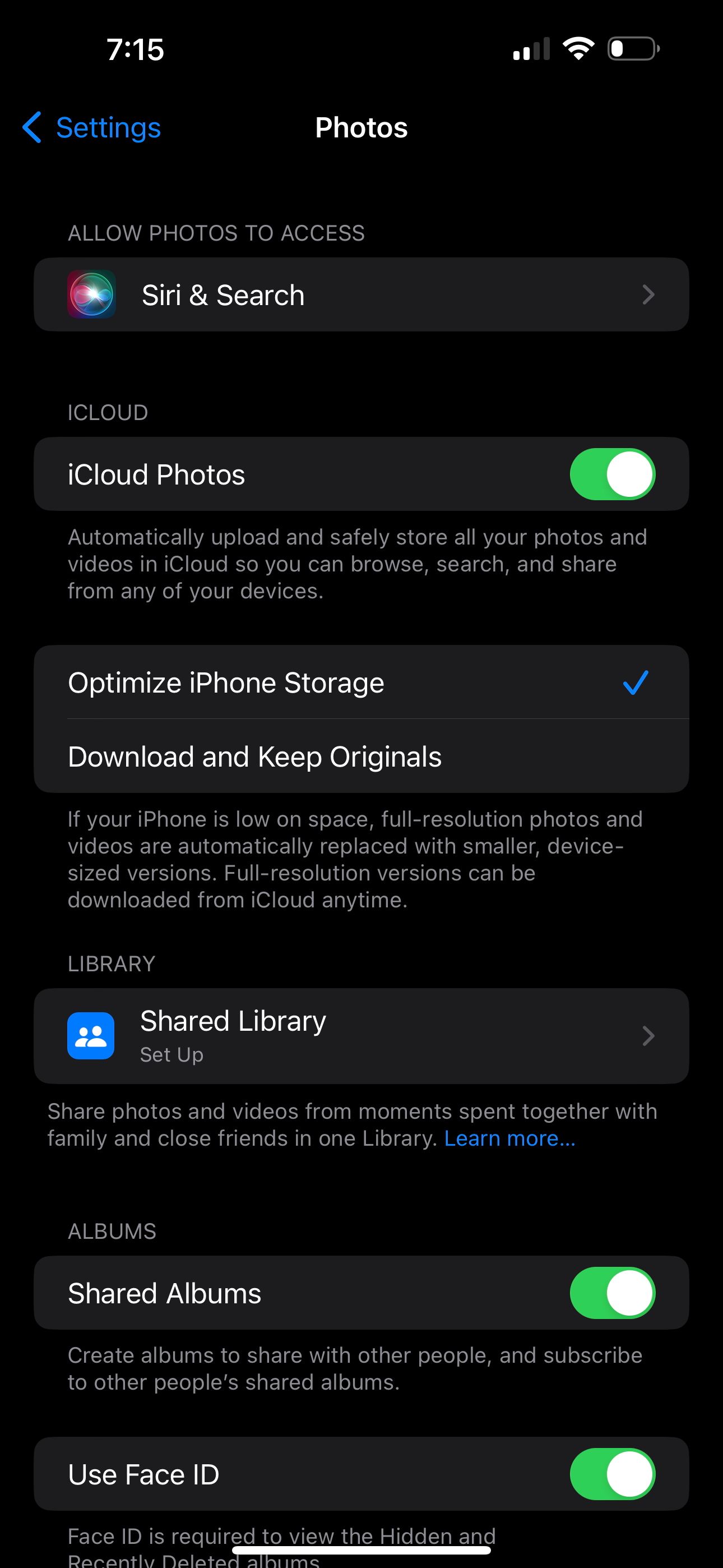Here's a detailed and cleaned-up caption for the image described:

---

The image depicts the "Settings" screen of a phone with a black background. At the top left, the time is shown as 7:15 in white text, while the top right displays two signal bars, three volume bars, and a battery icon with about 25% remaining. Centrally positioned at the top, "Photos" is written in white, and to the left, "Settings" is displayed in blue with a left-pointing arrow.

Below, there is a section titled "Allow Photos to Access." The first dark gray banner features "Siri & Search" in white text, accompanied by a colorful neon circle incorporating shades of purple, pink, green, and blue. The next item, "iCloud," appears in gray text.

A subsequent dark gray banner reads "iCloud Photos" in white with a green and white toggle switch indicating it's activated. Under this banner, a description states, "Automatically upload and safely store all your photos and videos in iCloud so you can browse, search, and share from any of your devices."

Two adjacent dark gray banners highlight "Optimize iPhone Storage" with a blue check mark and "Download and Keep Originals" in white text. Beneath these, in gray text against the black background, it reads, "If your iPhone is low on space, full-resolution photos and videos are automatically replaced with smaller device-sized versions. Full-resolution versions can be downloaded from iCloud anytime."

Moving to the next section labeled "Library," there is a dark gray banner stating "Shared Library" with a blue square icon featuring two people icons and the "Setup" option indicated by a right-pointing arrow. Below in gray text, it says, "Share photos and videos from moments spent together with family and close friends in one library," with a blue "Learn More..." link.

Following this, under the "Albums" section, a dark gray banner mentions "Shared Albums" with a green and white toggle switch turned on. It explains, "Create albums to share with other people and subscribe to other people's shared albums."

Finally, the last dark gray banner reads "Use Face ID" with the toggle switch on. Below it, in gray text, it mentions, "Face ID is required to view hidden and recently deleted albums." There is a white line under "to view hidden and," after which the text is cut off.